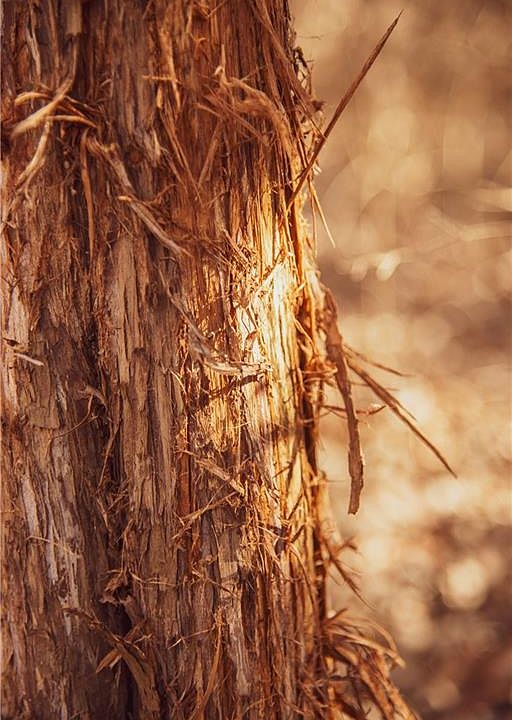This photographic close-up image captures the trunk of a tree outdoors, with a focus on its intriguing texture. The bark appears to be peeled off, exposing a network of stringy, straw-like fibers that dangle in various directions and resemble thin hair. These fibers are a soft caramel or bright golden brown color, adding a warm tone to the composition. Nestled among the fibers, a brown insect, camouflaged by its similarity to the filaments, is faintly visible with a distinct head and tail. Sunlight dapples the scene, primarily illuminating the middle of the trunk, creating a pronounced contrast with the out-of-focus, dark brown and tan background that appears to include more trees and foliage. The entire scene is void of any text, emphasizing the natural elements and textures.